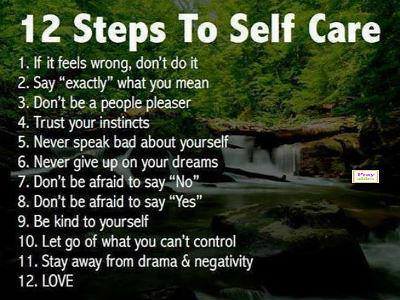The image features a serene outdoor scene with a lush forest of green trees and a small, cascading waterfall that deposits white water into a river below. Overlaid on this picturesque background, large white text spans the top, reading "12 Steps to Self-Care." Beneath this heading, a numbered list in smaller white text presents the steps:

1. If it feels wrong, don't do it.
2. Say exactly what you mean.
3. Don't be a people pleaser.
4. Trust your instincts.
5. Never speak bad about yourself.
6. Never give up on your dreams.
7. Don't be afraid to say no.
8. Don't be afraid to say yes.
9. Be kind to yourself.
10. Let go of what you cannot control.
11. Stay away from drama and negativity.
12. Love.